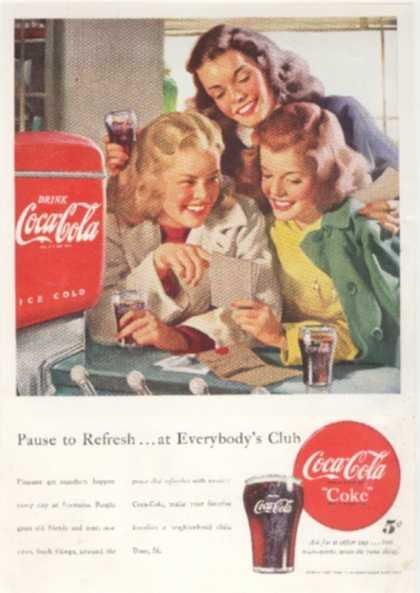This full-page, color advertisement from the 1950s or 1960s showcases a vintage Coca-Cola scene. The top half features an illustration of three young women at a classic soda fountain bar. Two of the women are seated, while one stands behind them, all sporting 1950s-style short and wavy haircuts. The standing woman is leaning over, holding a glass of Coca-Cola in one hand and what appears to be a photo in the other. The seated women are engaged with a stack of photos; one, dressed in yellow and green with red hair, is holding the photos, while the other, in a white jacket with blonde hair, holds a glass of Coke. They all display warm, joyful smiles as they interact with the photos. On the left side of the image, there is a distinctive red, rounded rectangular cooler or soda fountain with the Coca-Cola logo. Below the illustration, the text reads, "Pause to refresh at everybody's club." Accompanying this text is a red circle with the Coca-Cola logo and an image of a glass of Coca-Cola, labeled as "Coke" and priced at five cents. The advertisement radiates a nostalgic and inviting atmosphere, encouraging viewers to enjoy a refreshing Coca-Cola.